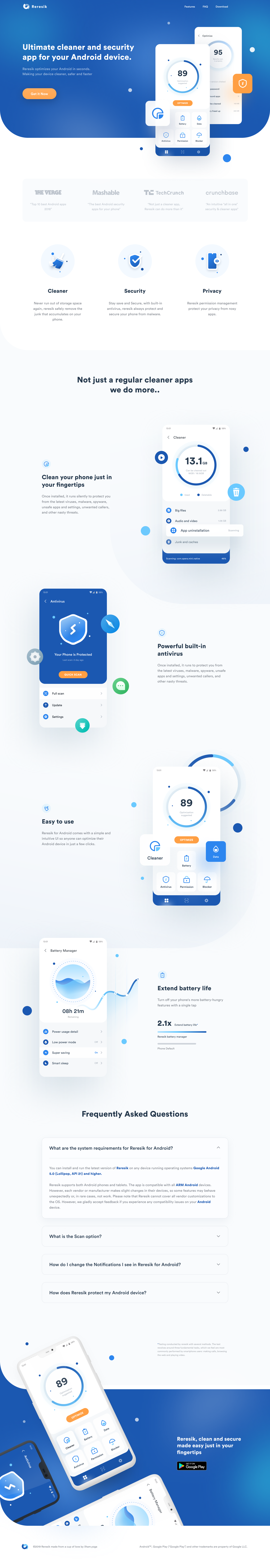This image is a blurry screenshot of a promotional display for an Android security and cleaner app. The top section features a blue bar with the app’s name: "Ultimate Cleaner and Security App for Your Android Device." Below this, an interface display shows the number "89" inside a circle with several icons underneath. Further down, the number "95" is seen with some text written below it.

The main content is divided into six sections titled: "The Verge," "Mashable," "TechCrunch," "Crunchbase," "Cleaner," and "Security." Each section appears to have descriptions or testimonials.

A prominent tagline reads: "Not just a regular cleaner app, we do more. Clean your phone with just your fingertips," followed by a paragraph of explanation. 

On the right side, there's a white rectangular box featuring a "13.1" in a circle, outlined in blue. Adjacent to it is a blue box. Text beside it reads, "Powerful built-in antivirus." Below this, the text "Easy to use" can be seen alongside icons labeled "Cleaner" and other functions that are not legible due to the image quality.

Further down, a circle with a blue wave graphic displays "Battery Manager" and "08h 21m," indicating 8 hours and 21 minutes of battery life remaining. Additional text mentions extending battery life. "2.1x" is shown, possibly indicating a performance metric.

A segment titled "Frequently Asked Questions" is visible, with one expanded question reading, "What are the system requirements for R-E-S-R-E-R-E-S-I-K for Android?" Accompanying this is a paragraph discussing Android requirements, though it’s not fully readable. Three more dropdown questions are listed: "What is the scan option?", "How do I change the notifications for Android?", and "How does R-E-S-R-E-R-E-S-I-K protect my Android device?"

At the bottom, there’s a visual of a phone screen within a blue box area and a Google Play Store link for downloading the app.